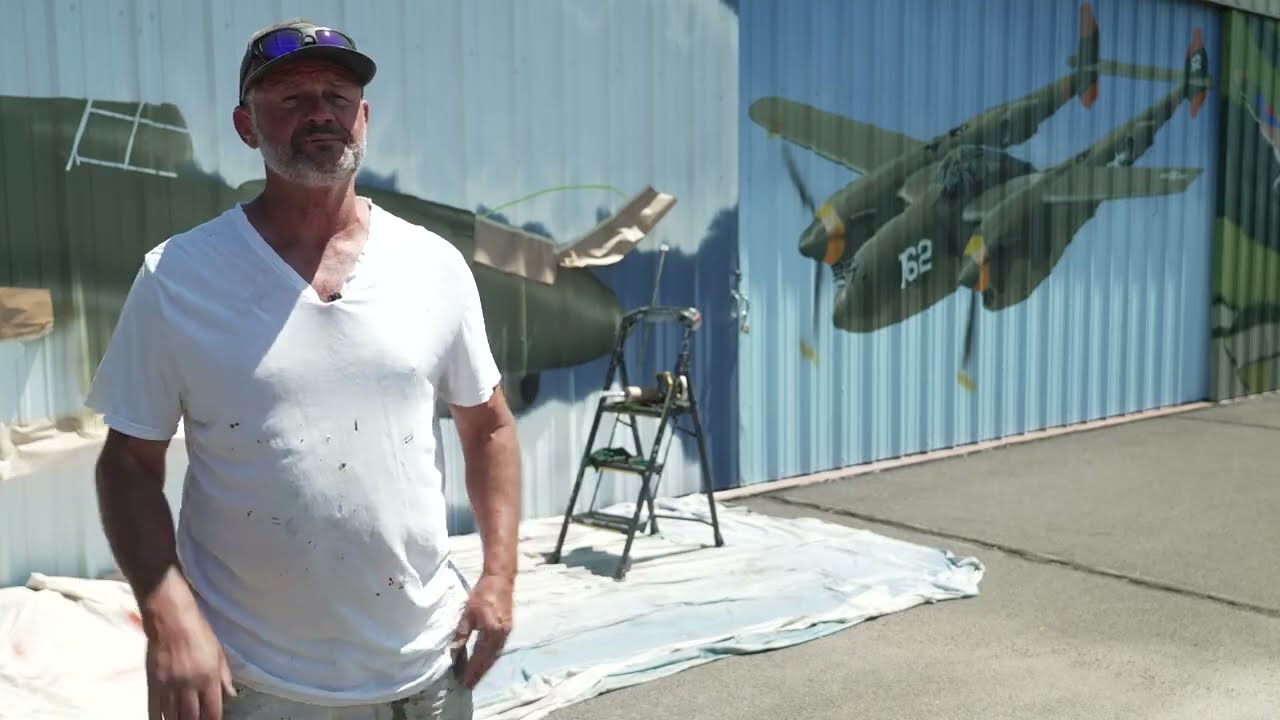In this image, a larger, older Caucasian male, possibly middle-aged, is standing on the left side. He sports a gray and white beard and mustache, and wears a white V-neck t-shirt that appears slightly dirty, along with a baseball cap adorned with sunglasses perched on its bill. His hands are casually in his pockets, giving the impression he might be in the middle of an interview.

Behind him, he seems responsible for painting vibrant murals of World War II planes on the large metal doors, characteristic of those found in storage facilities or airplane hangars. To the right, a finished mural depicts an olive green fighter plane with the number 162 clearly visible, soaring against a backdrop of a blue sky. Directly behind him, another similar mural appears in progress, suggesting he is still working on it. In this painting area, a stepladder and a white drop cloth are prominently placed, hinting at his meticulous approach to keeping the workspace clean. The scene emanates a sense of dedication and artistry, capturing a historical moment in vivid detail.